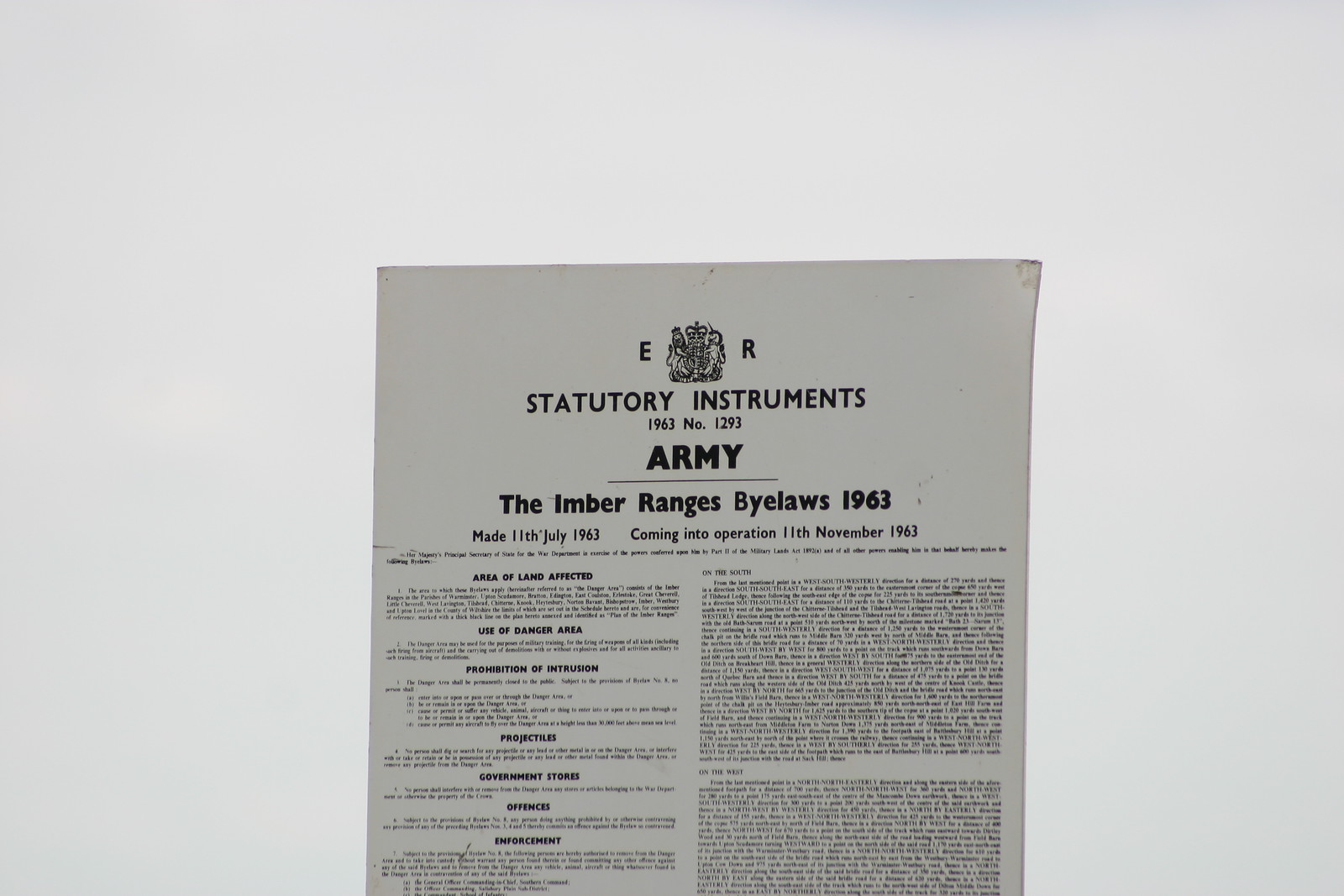A piece of paper, likely a formal document or poster, sits on a white surface. It displays a detailed crest featuring a lion on the left, a unicorn on the right, and a crowned shield in the center. To the left of the crest is the letter "E" and to the right, the letter "R". Below the crest, the title reads, "Statutory Instruments," followed by the subtitle, "1963, Number 1293". The document is titled "Army, The Ember Ranges Bylaws, 1963," with details indicating it was made on 11th July 1963 and came into operation on 11th November 1963. Various sections are labeled with headings such as "Area of Land Affected," "Use of Danger Area," "Prohibition or Intrusion," "Projectiles," "Government Stores," "Offenses," and "Enforcement." The text, mostly black on white, contains both legible and illegible portions, with much of it in small print. The overall background is plain and white.